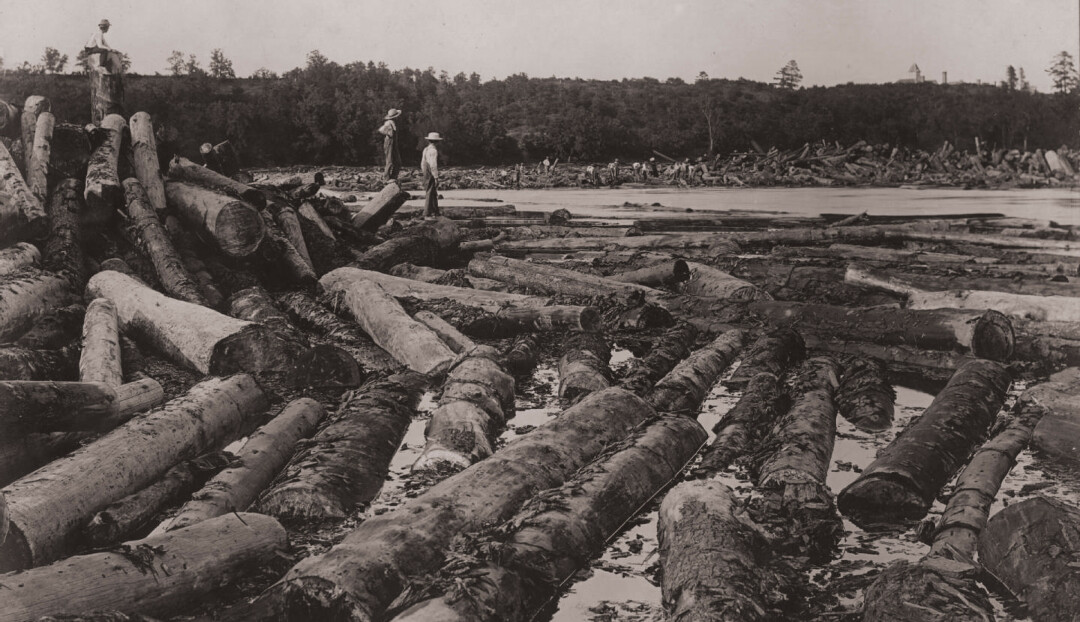This vintage black-and-white photograph captures a desolate logging operation on what appears to be the dried-out shore of the Chippewa River. The sky is overcast, painting a gray backdrop for a scene filled with somber hues. Stretching from right to left across the image is a dense forest, giving way to a clutter of felled logs scattered haphazardly along the shore and shallow, swampy waters. In the lower third of the image, logs are piled as high as five feet in some areas, spilling into the water where they float at various angles. Two lone figures, possibly children or young workers, stand on the shore with their backs to the camera, gazing into the distance. They wear overalls and hats, adding to the rustic ambiance of the scene. Just above them, on the left side, another figure sits atop a log, observing the two below. The photograph, rich in historical context, portrays not just the labor-intensive nature of the logging industry but also a poignant moment within a barren, log-cluttered landscape.